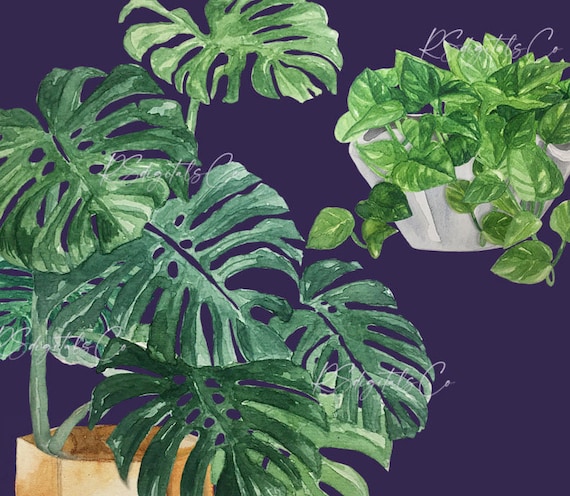The image depicts a detailed painting of various potted plants set against a deep purple background. In the bottom left-hand corner, a brownish plant pot hosts a vibrant green plant with seven large, palm-like leaves. These leaves are distinctive, characterized by their segmented structure and wide openings along the middle line. Some leaves reach upwards while others cascade downwards towards the right side of the painting. In the upper right-hand corner of the artwork, a white, circular pot contains a green ivy-style plant whose delicate tendrils spill over the edges and drape downward. Additionally, there is a cream-colored pot with a plant resembling a fern, featuring broad leaves with holes. White cursive text, although somewhat obscured by the plant foliage, includes an artist's signature, reading "RSGOTALS," with the initials "ROG" discernible in the top-right corner. The composition features a harmonious blend of green, white, brown, and light gray colors against the rich, dark blue-purple backdrop.